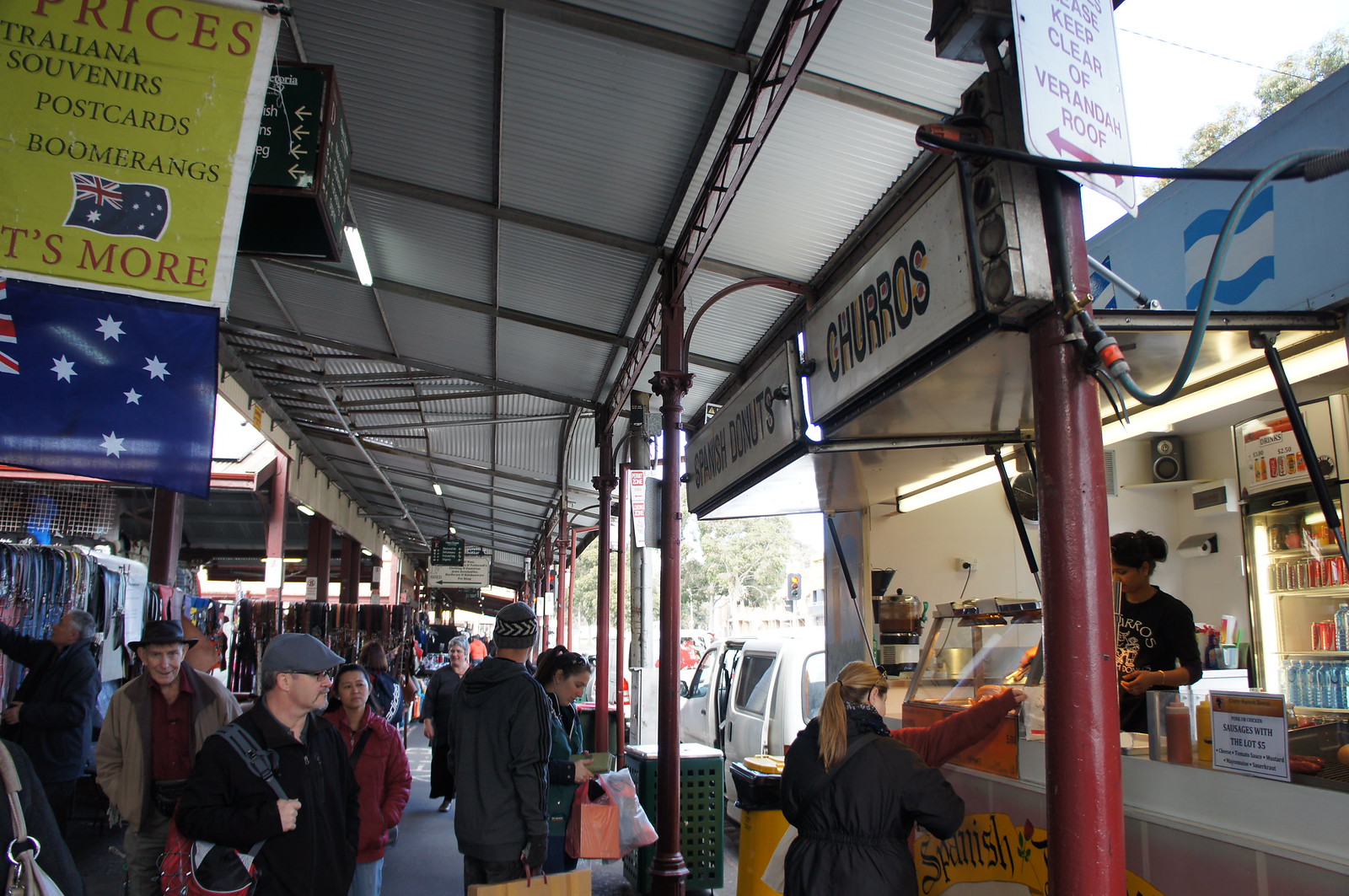The photograph depicts a bustling scene under a large, diagonally-sloped, metal-roofed pavilion supported by red and copper-colored poles. Several people clad in winter clothing are lined up in front of a food stand that prominently advertises "Churros" and "Spanish Doughnuts" on white signs. The stand is operated by a dark-skinned woman working behind the counter, with shelves stocked with canned goods and kitchen machinery visible in the background against a white wall. The diverse crowd includes a man wearing a black jacket with a bag slung over his shoulder, a woman in a red jacket, and an Asian woman among others. In the upper left corner of the image, a partially visible sign reads "Australiana, Souvenirs, Postcards, Boomerangs" alongside an Australian flag. Further into the scene, other people can be seen perusing various displays. A street sign nearby cautions to "Keep Clear of Veranda Roof," marked by a red arrow.